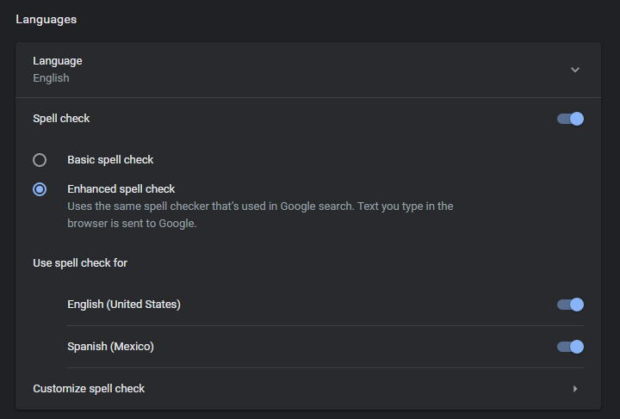The image showcases a detailed view of a language and spell check settings menu within a document editing interface. The top section is a black banner with the heading "Languages" prominently displayed in white text. Beneath this, a slightly lighter black overlay houses a series of settings.

The first setting is labeled "Language" in bold white text. Directly below this, "English" is displayed with a drop-down arrow indicating more language options.

The next section is dedicated to spell check settings. The main spell check toggle is slid to the right, indicating that spell check is enabled. There are two spell check options available: "Basic Spell Check" and "Enhanced Spell Check." The latter is currently selected, as evidenced by a blue filled-in button next to its name. A brief description notes that this setting utilizes the same spell checker used in Google Search.

Below this, another setting shows options for using spell check for multiple languages. Both "English" and "Spanish" are listed, with toggles next to each slid to the right to show they are active.

Finally, there is an option labeled "Customize Spell Check," though no specific details are provided for this setting.

The entire interface is separated by thin lines dividing each section, and the text is neatly organized to enhance readability against the dark background.